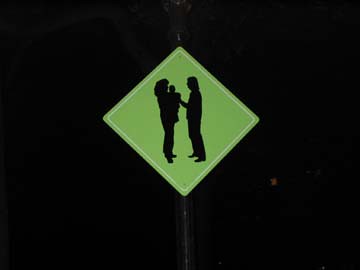This color photograph, taken at night, features a diamond-shaped, light green street sign, centrally positioned in the frame against a black background. The sign has a thin white border around its inner edge and is mounted on a slightly scraped black metal pole. Within the sign, a couple is depicted standing upright. The woman, positioned on the left, faces the man and stands with her right foot extended to the side. She is holding a baby in her arms. The man, on the right, stands with his feet pointed towards the woman, extending his right arm to touch the baby. The overall scene suggests a moment of intimate interaction captured and symbolized on the street sign.